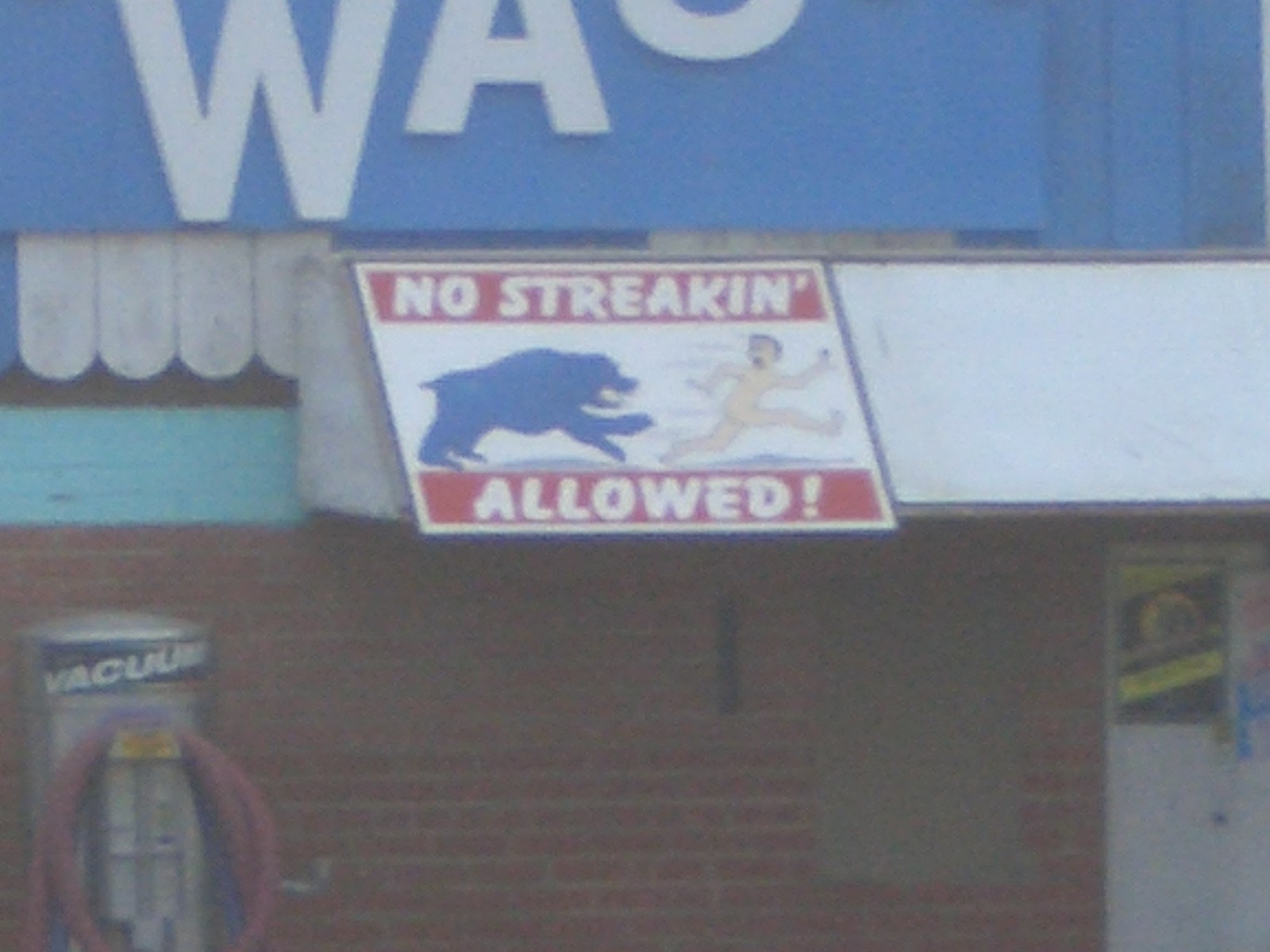The image depicts the exterior of a car wash building constructed from red brick. The photograph captures primarily the first floor, prominently featuring a white entrance door. To the left of the door, a vacuum cleaner with a coiled red hose is mounted and ready for use. Above the entrance, a white canopy extends outward, supporting a humorous warning sign. This sign is bordered by red bands at the top and bottom and declares "No Streaking Allowed" in bold white letters. The central portion of the sign humorously illustrates a naked man fleeing from a blue bear. Additionally, a partial view of the car wash's main signage is visible, showcasing a blue background with fragmentary white text, suggesting the word "Wash."